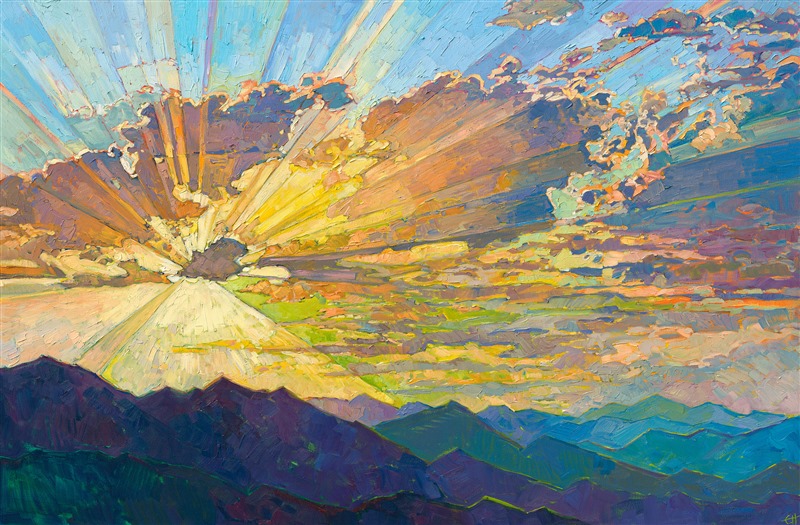This piece is a textured painting, possibly oil or watercolor, capturing a breathtaking landscape during a sunrise or sunset. The scene is dominated by a dynamic and busy sky, rich in gradient hues that shift from light blue to mottled stripes of blues, reds, violets, and orange-yellows towards the right. The focal point is a large, resplendent cloud cluster in the center, with shades transitioning from yellow to tan to orange to rust. Hidden behind these clouds, the sun sends out radiant beams of light in light white, gray, pink, and green. The upper portion of the sky shows a purer blue amidst the diverse pastel tones. Below this luminous sky, a multicolored mountain range spans the bottom of the painting, with peaks in silhouette illuminated by the sun. The mountains start off dark and become progressively lighter, transitioning through bluish purple, green, teal, and aqua hues. The textured brushstrokes and the play of light across the entire composition create a vivid portrayal of natural beauty.